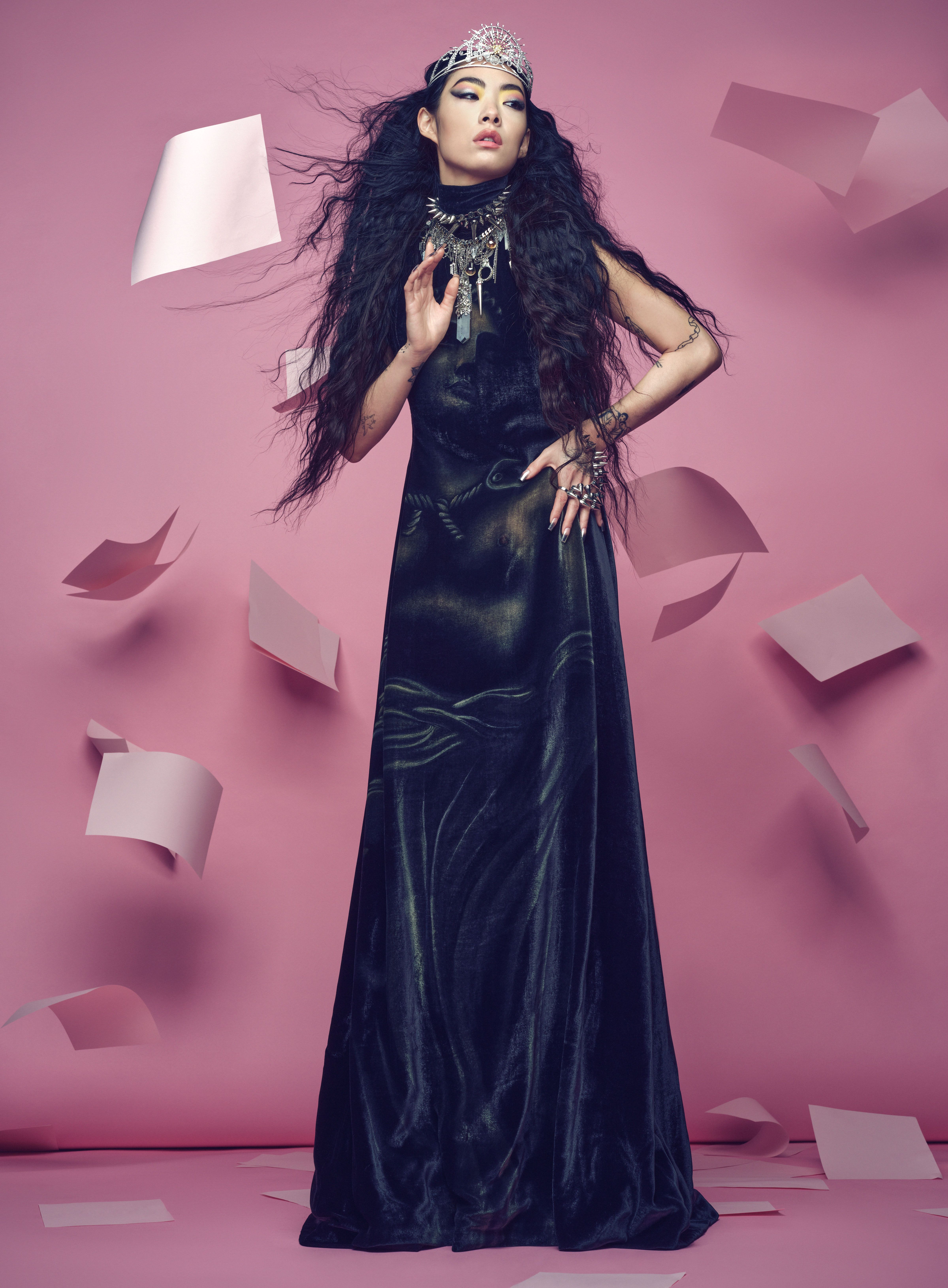The photograph features an Asian woman with long, flowing black hair that appears slightly messy and is being blown outward, suggesting the presence of wind or a fan. She is adorned with a silver crown and some gold elements, resembling a princess crown, emphasizing a regal aesthetic. Her outfit is a sleeveless, long black dress that extends past her feet, obscuring them from view. The dress has a gothic flair, accented with ropes. The woman has black tattoos on her arms, and she accessorizes heavily with jewelry, including multiple rings on her left hand and a large silver and gold necklace around her neck. Her right arm is bent with her hand on her hip, while her left hand is touching the necklaces. The background is entirely pink, with pink flooring and pink sheets of paper floating in the air, adding to the dynamic, windblown effect of the scene.